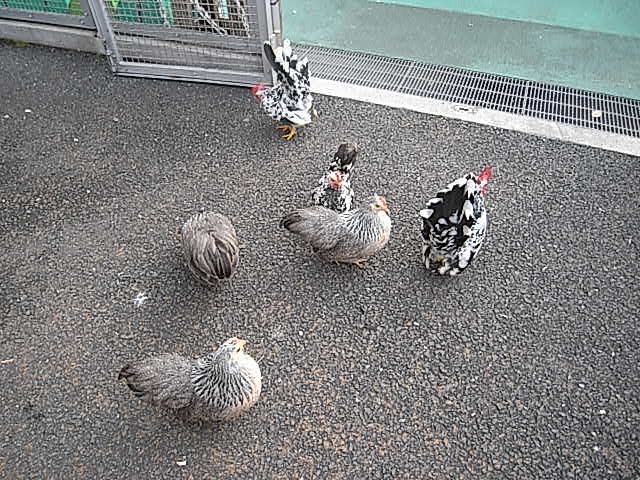The image depicts six chickens on a stony, gravel-like ground. Three of the chickens are plump with gray and black feathers, and the other three display a distinct black and white feather pattern. All the chickens have yellow beaks and feet, along with a small red comb on the top of their heads. The scene includes a background with a metal grating featuring holes and a nearby open metal door. The chickens appear to be casually walking around and are closer in the foreground, with the gray ones being more prominent. The setting is ambiguous, possibly a farmyard or a similar environment.